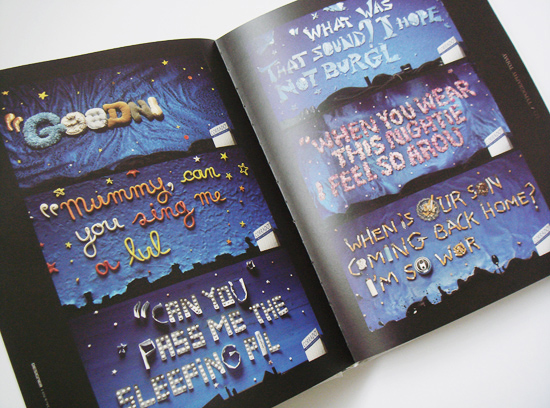This image depicts an open black book resting on a pristine white table. Each page of the book features three rectangular sections with a uniform blue background. These rectangular sections contain text and are adorned with star patterns.

On the left page, the top rectangle bears the phrase, "Good and I." The middle rectangle reads, "Mummy, can you sing me a lull?" The bottom rectangle displays the text, "Can you press, can you pass me the sleeping pill?" 

On the right page, the top rectangle states, "What was that sound? I hope not bird." The middle rectangle contains the message, "When you wear this nightie, I feel so arow." The bottom rectangle reads, "When is our sun coming back? We'll worry."